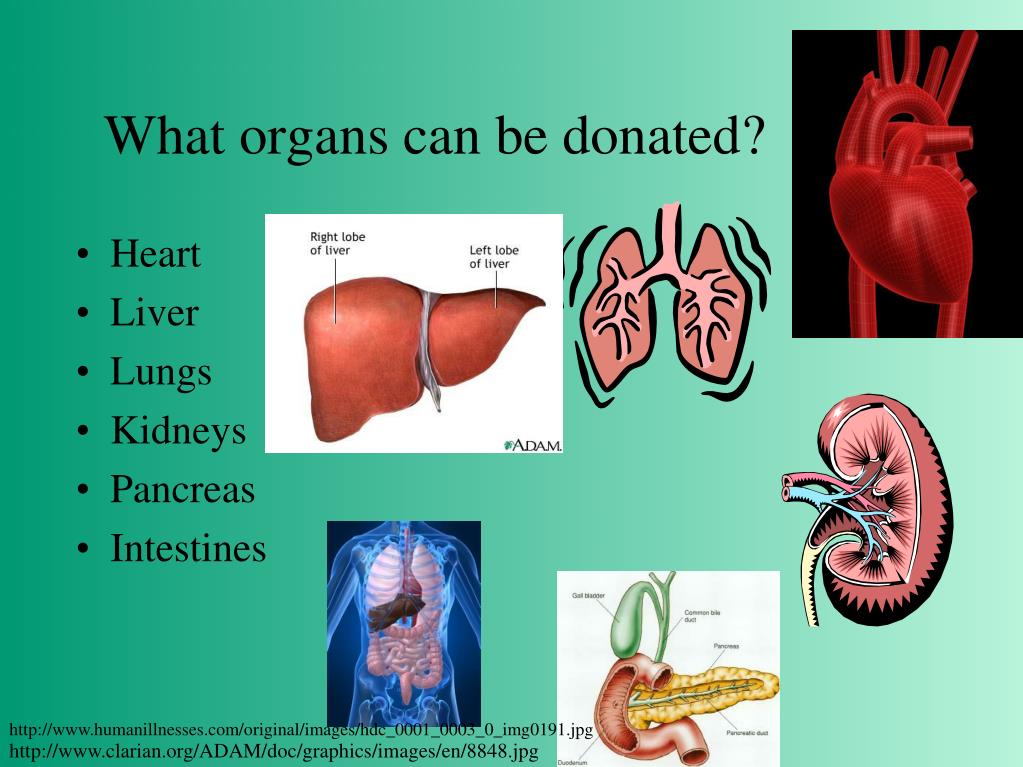The illustration designed for a PowerPoint slide focuses on the topic of organ donation and comes with a green background. Across the top of the slide, the phrase "what organs can be donated?" is prominently displayed in black letters with only the 'W' capitalized. On the left-hand side, there is a bulleted list of organs that can be donated: heart, liver, lungs, kidneys, pancreas, and intestines. 

Adjacent to this list, there are corresponding thumbnail-sized images illustrating these organs. The heart image is particularly notable, depicted in red against a black background. Directly below the text, there's a detailed anatomical illustration of a liver, with clearly labeled sections indicating the right and left lobes. Nearby, an image of the complete digestive system provides further anatomical context. Additional illustrations include a pair of lungs shown to the right of the liver, each depicted with labeled lines. Along the bottom left corner, small print credits attribute the sources of these images. Overall, the slide effectively combines textual and visual elements to convey information on organ donation.